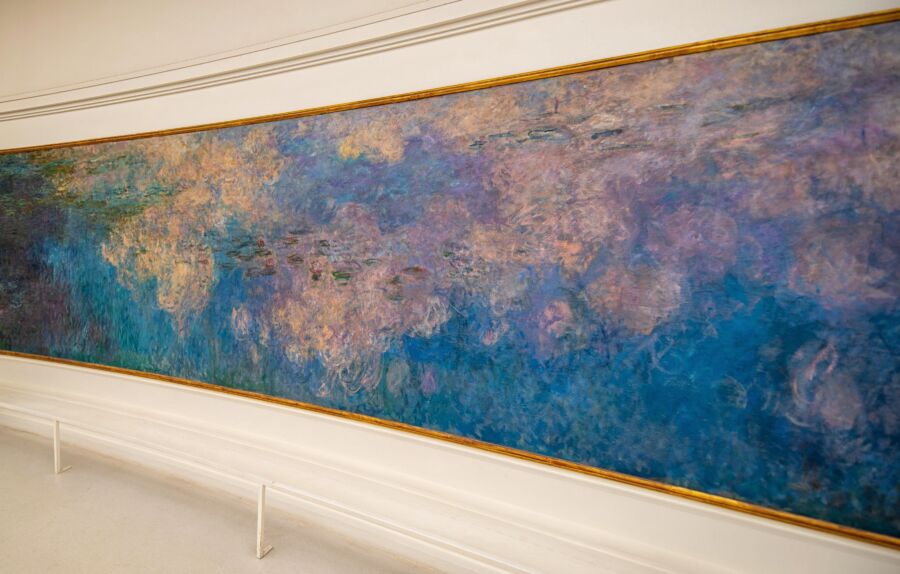The image depicts a very large, impressionistic oil painting that spans across a curved white wall, potentially extending at least 10 feet in length. The painting features an array of colors, predominantly blue, white, magenta, and green, creating a scene that is open to interpretation, possibly representing a body of water with fish and coral, reflecting pink and white clouds. The artwork is bordered by a golden frame along the top and bottom edges and is elevated above a very light gray floor, just beneath a white ceiling. A small white railing runs from the bottom middle of the picture upward and to the left, presumably to keep viewers at a respectful distance from the mural.